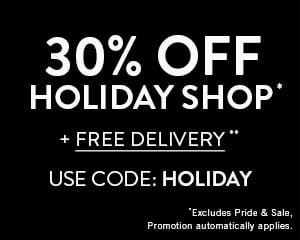The image features a black rectangular background with a clear, bold promotional message. At the top, large white bold letters announce "30% OFF". Just below, in slightly smaller but still bold white letters, it reads "HOLIDAY SHOP" with an asterisk (*) to the right. Below this, in smaller capitalized white letters and underlined, it states "PLUS FREE DELIVERY" with two asterisks (**) to the right. Further down, in bold white capital letters, the instruction "USE CODE: HOLIDAY" is prominently displayed. At the very bottom, in much smaller white text, a disclaimer reads "* Excludes Pride as sale promotion automatically applies." The rest of the image consists of empty black space, particularly around the edges and at the top, enhancing the visibility of the text.